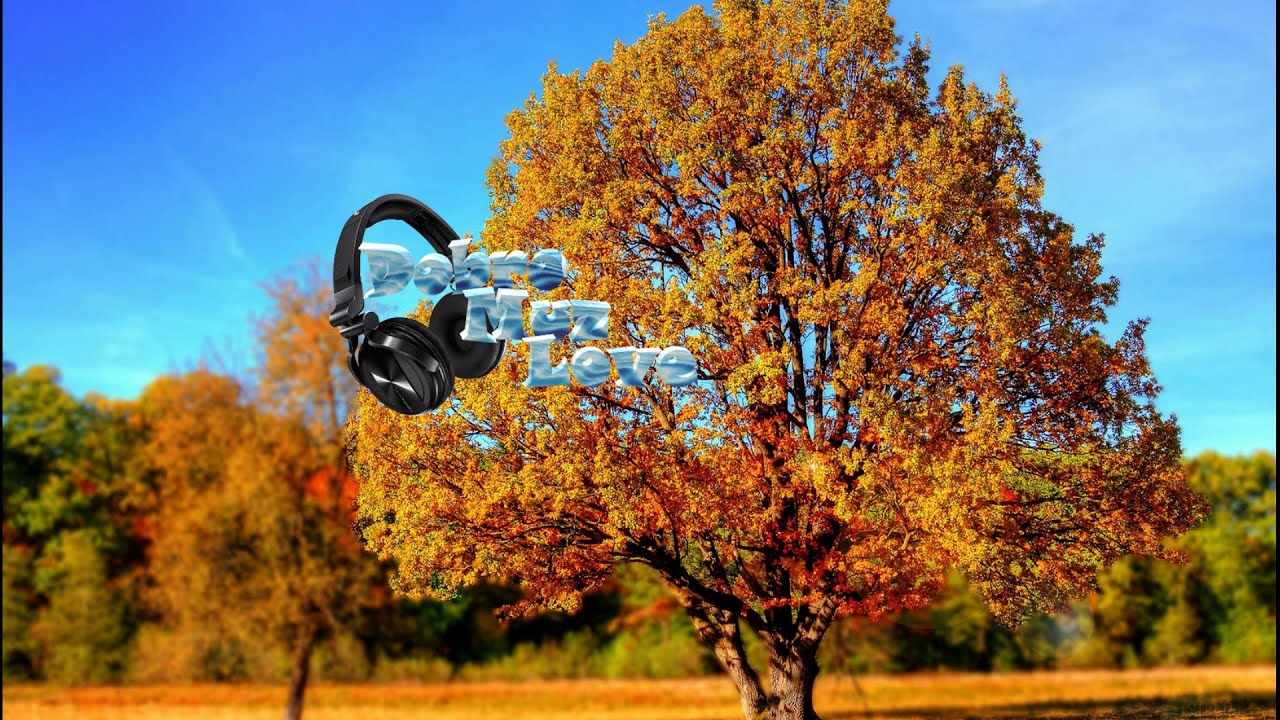This image captures a picturesque autumn scene with vibrant fall foliage. The centerpiece is a large tree whose leaves are ablaze in shades of yellow, red, and orange, signifying the peak of the fall season, likely around September to November. The crown of the tree dominates the image, with thin branches interspersed among the colorful leaves, while only a small part of the trunk is visible at the bottom. Surrounding this striking tree are several other trees, blurred in the background, displaying similar autumnal hues of yellow and orange. Above, a clear blue sky stretches without any clouds, adding to the serene atmosphere. Superimposed in the middle of the image, slightly to the left, is an edited graphic featuring black headphones and the text “Debra Much Love” written in green and blue. This text is vertically stacked and adds a modern touch to the otherwise natural and timeless scene.